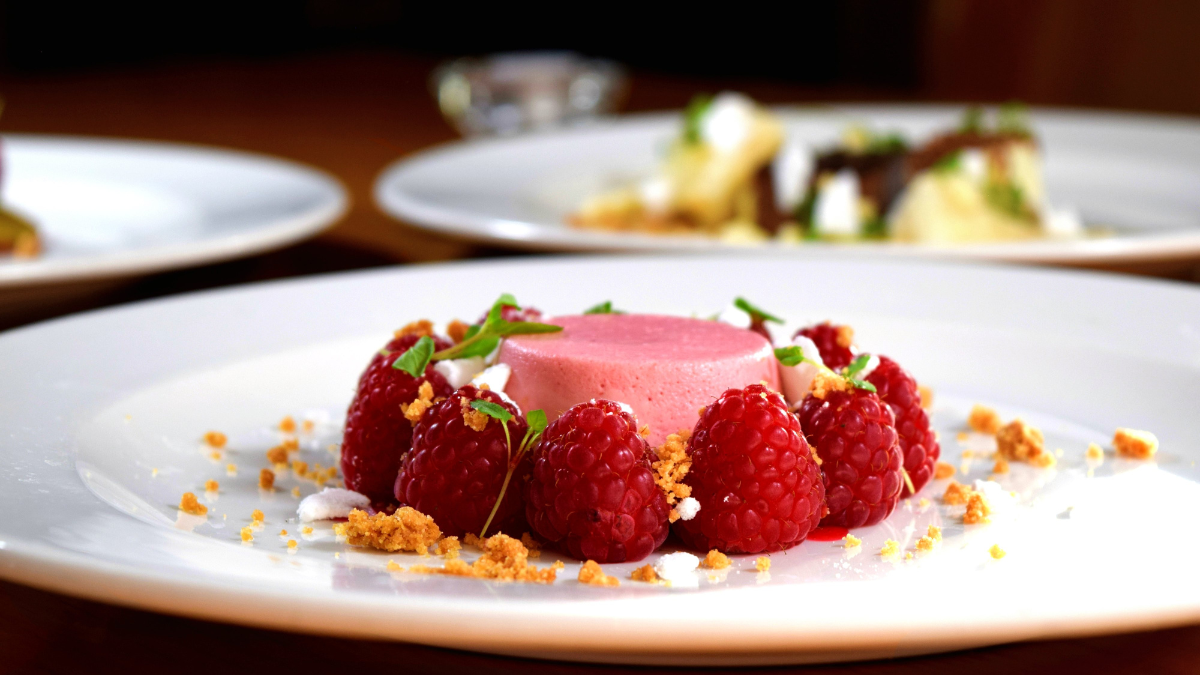This image showcases a beautifully plated raspberry mousse dessert on a large white dinner plate. The mousse, appearing gelatinous and foamy with a rich reddish-pink hue, is shaped into a cup-like formation and positioned upside down in the center of the plate. It is elegantly surrounded by approximately twelve vibrant red raspberries, accented with sprigs of microgreens. An artful dusting of ground cinnamon and sugar encircles the mousse, adding a touch of warmth and contrast. Further enhancing the presentation, dollops of white cream are also present on the plate. In the blurry background, a secondary dessert can be seen, predominantly white with what appears to be a drizzle of chocolate sauce and garnished with green herbs or decorative sprinkles, all set against a dark brown wooden table. Additional blurred white plates with unidentifiable food elements are partially visible, contributing to the sophisticated and inviting dining scene.